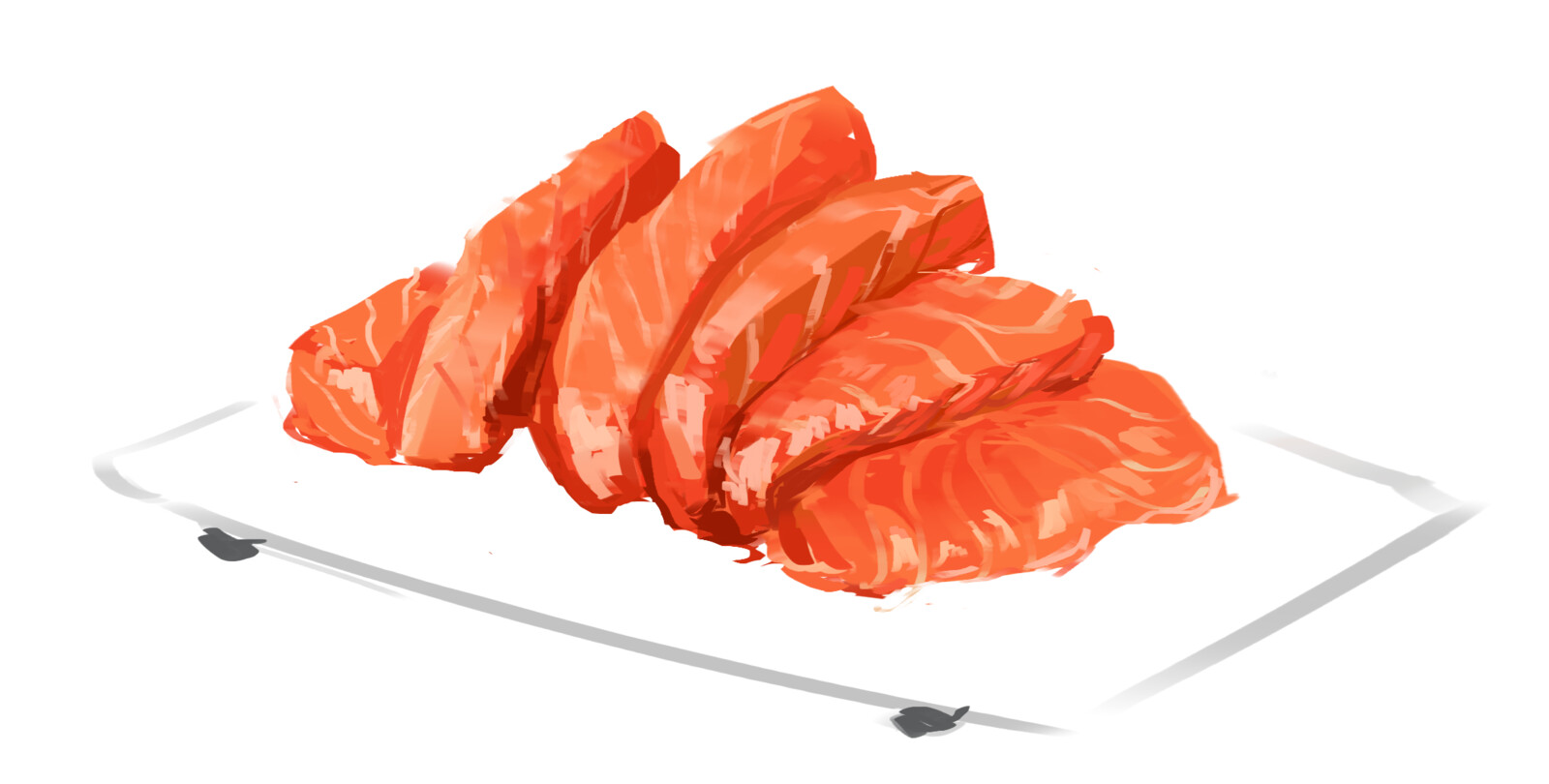The image depicts a detailed, cartoon-like illustration of six thick but thinly sliced pieces of raw salmon arranged on a white cutting board with black feet underneath it. The salmon slices, characterized by their salmon pink color interspersed with white squiggly lines, are stacked both horizontally and vertically, with some pieces lying flat while others are bunched together and standing upright. The white cutting board features a silver border with a sheen, adding a reflective quality to its appearance. Despite resembling clip art, the image retains a slightly realistic touch in its representation of the fish. The overall scene appears simplistic but carefully crafted, potentially set in a kitchen environment.